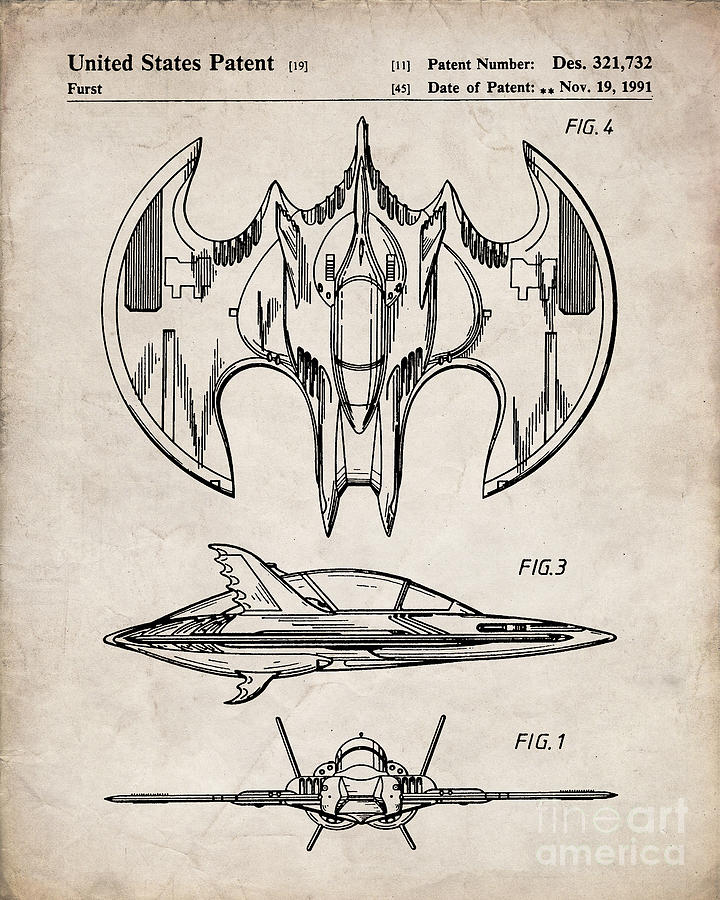This hand-drawn sketch appears on aged, yellow parchment and details a design reminiscent of the Batplane from comic books, as indicated by the stylized features and the inscription "United States Patent 19,” with the patent number DES321732 dated November 19, 1991. The drawing is labeled "Figure 4," "Figure 3," and "Figure 1," each offering different perspectives of the aircraft. Figure 4 shows a top-down view where the wings mimic the shape of a curved sword with a twin-tipped nose and a cockpit on top. Figure 3 gives a side profile, revealing the tapered nose, extended wings, and the streamlined rear. Figure 1 offers a head-on view, displaying the wings as lines and highlighting two stabilizers. The paper is marked with “Finite America” as a white watermark. The black ink used for the sketches contrasts with the yellowed paper, adding to the vintage aesthetic. This rendering appears to capture a futuristic aerial vehicle, possibly evoking elements of modern drones or UAPs, emphasizing its potential to be both a scientific marvel and a pop culture icon.